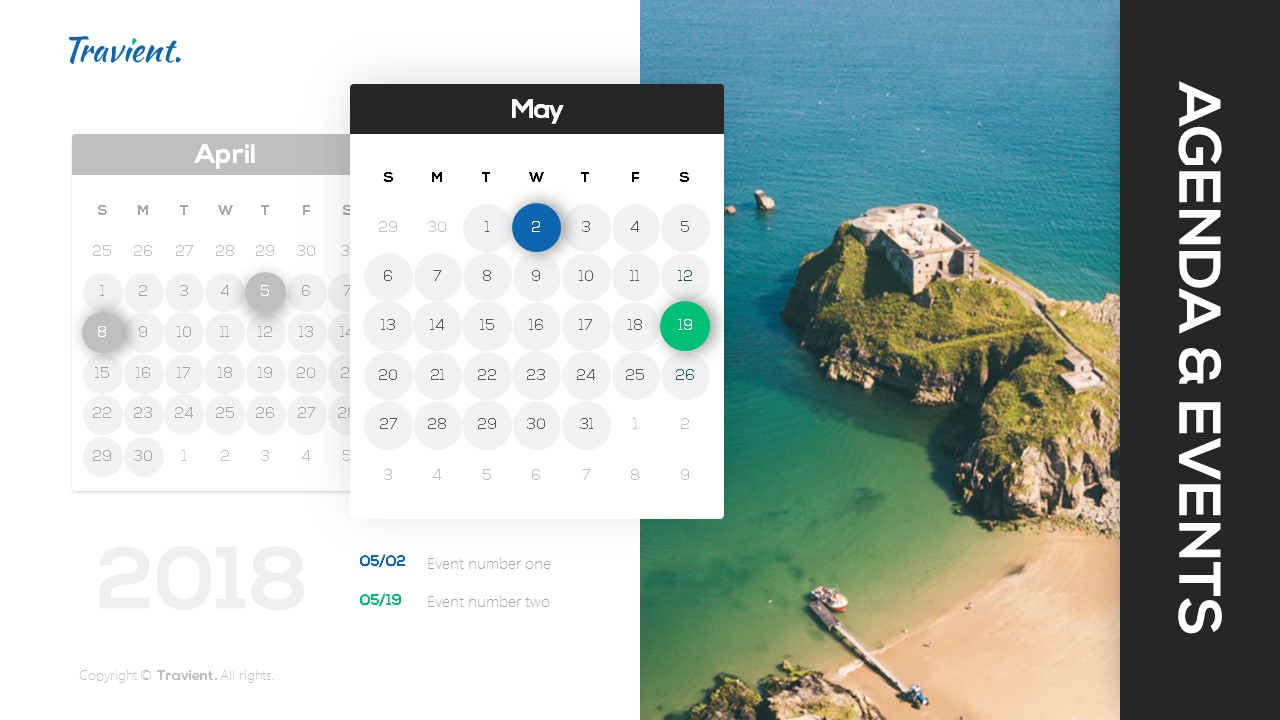The image depicts a section of a website named "Traviant," with its logo prominently displayed in blue text at the top left corner, punctuated by a small green dot over the 'i'. Below the logo, two overlapping calendar widgets are visible. The first calendar, representing April 2008, is grayed out with specific dates, April 5th and April 8th, marked in gray. This calendar is slightly obscured by the second calendar for May 2008, which is brought to the foreground with a white background and black text. Each day on the May calendar is circled, with April 2nd distinguished by a dark blue circle and a white '2' in the center, and April 19th highlighted by a green circle containing a white '19'. Below the calendars, "2018" is noted, possibly indicating a current event or reference year.

To the right of the calendars, text entries labeled "502" for May 2nd and "519" for May 19th list "event number one" and "event number two," respectively. Adjacent to these event details is an image of a fortress-like structure built on rocky outcrops extending into a body of water. The rocks are topped with greenery and emerge directly from a beach. A smaller adjacent dock harbors a small white and red boat. Flanking this composition on the far right, a black vertical banner displays "Agenda and Events" in white text.